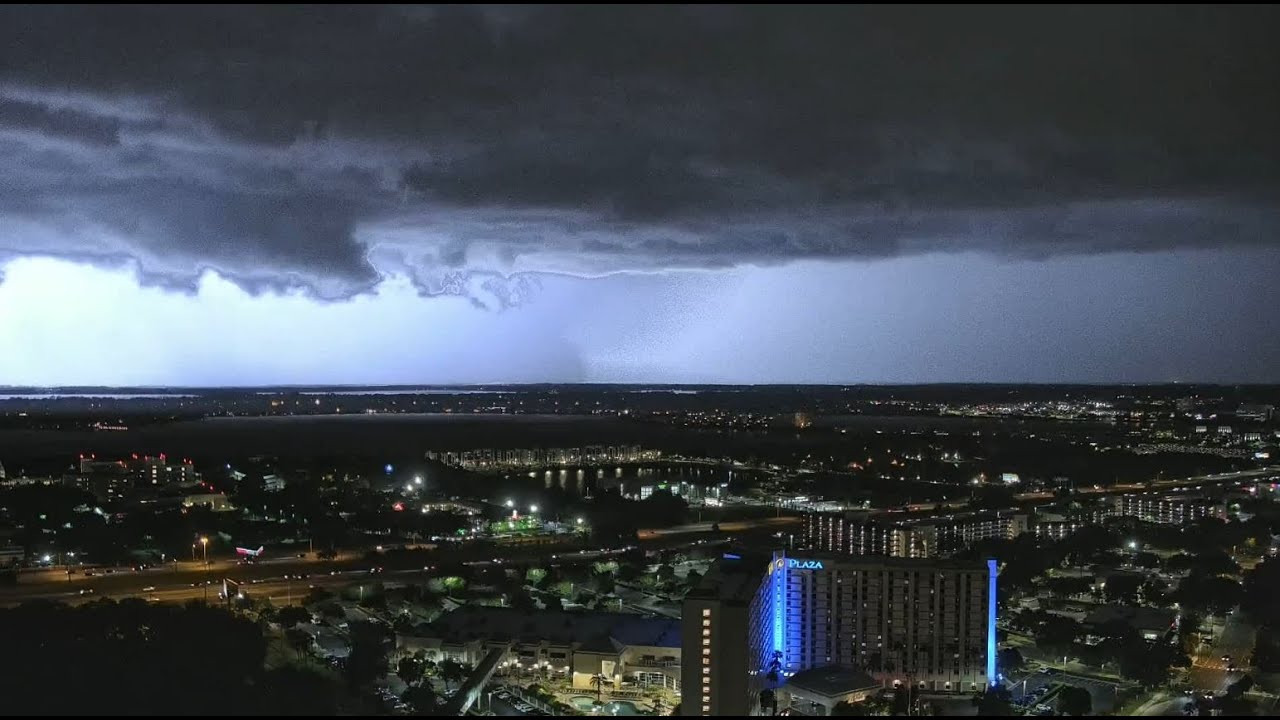This full-color aerial photograph captures a sprawling city poised on the brink of a fierce storm. Taken using both natural and artificial light, the image is a horizontally rectangular shot likely snapped from a drone or airplane, giving a bird’s eye view of the urban landscape. The city lies seemingly flat, possibly in a valley, and is reminiscent of Las Vegas with its vibrant and contrasting lighting against the impending gloom.

Dominating the composition are ominous dark clouds that blanket the top portion of the sky, signaling a deluge imminent. A particularly striking feature is a large building near the bottom center, lit up with blue neon lights and marked with the word "Plaza." This blue hue stands out as the primary color element in the otherwise muted, gray environment.

In the midst of the darkening cityscape, numerous buildings and streets are illuminated, revealing high-rise structures as well as smaller homes and apartments. The photograph reveals an eerie blend of tranquility and tension, with the city lights twinkling beneath an oncoming storm. The clouds appear to hang low, almost touching the skyline, and there’s even the suggestion of a tornado forming in the distance, heightening the sense of an impending natural upheaval.